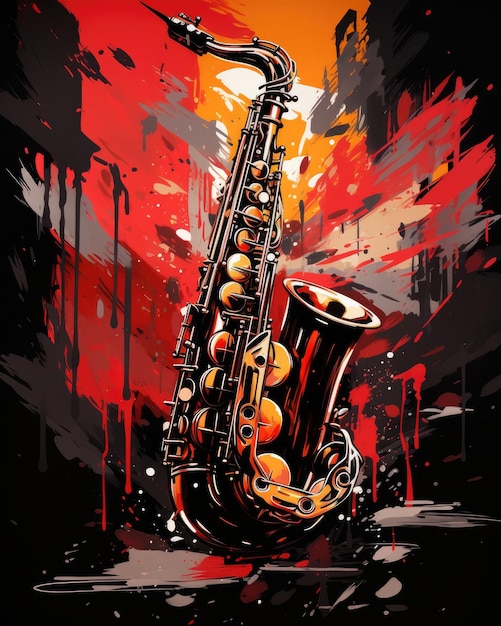The image is a tall, rectangular artwork dominated by a large golden saxophone, which takes up almost the entire height and width of the piece. The saxophone features graphic, reflective touches, showcasing lighter sections of shiny brass along with darker hues of red and black, likely reflections off its shiny exterior. The background is an abstract mix of colors, with a vibrant orange center surrounded by red, and bordered by darker shades of black and beige. The top incorporates blends of red, orange, white, and gray, with some of the colors appearing to bleed and run together, adding to the dynamic, fluid nature of the composition. The overall effect is that of a striking, visually compelling painting, or possibly a digital illustration, with the saxophone as the focal point against a vivid, abstract backdrop.